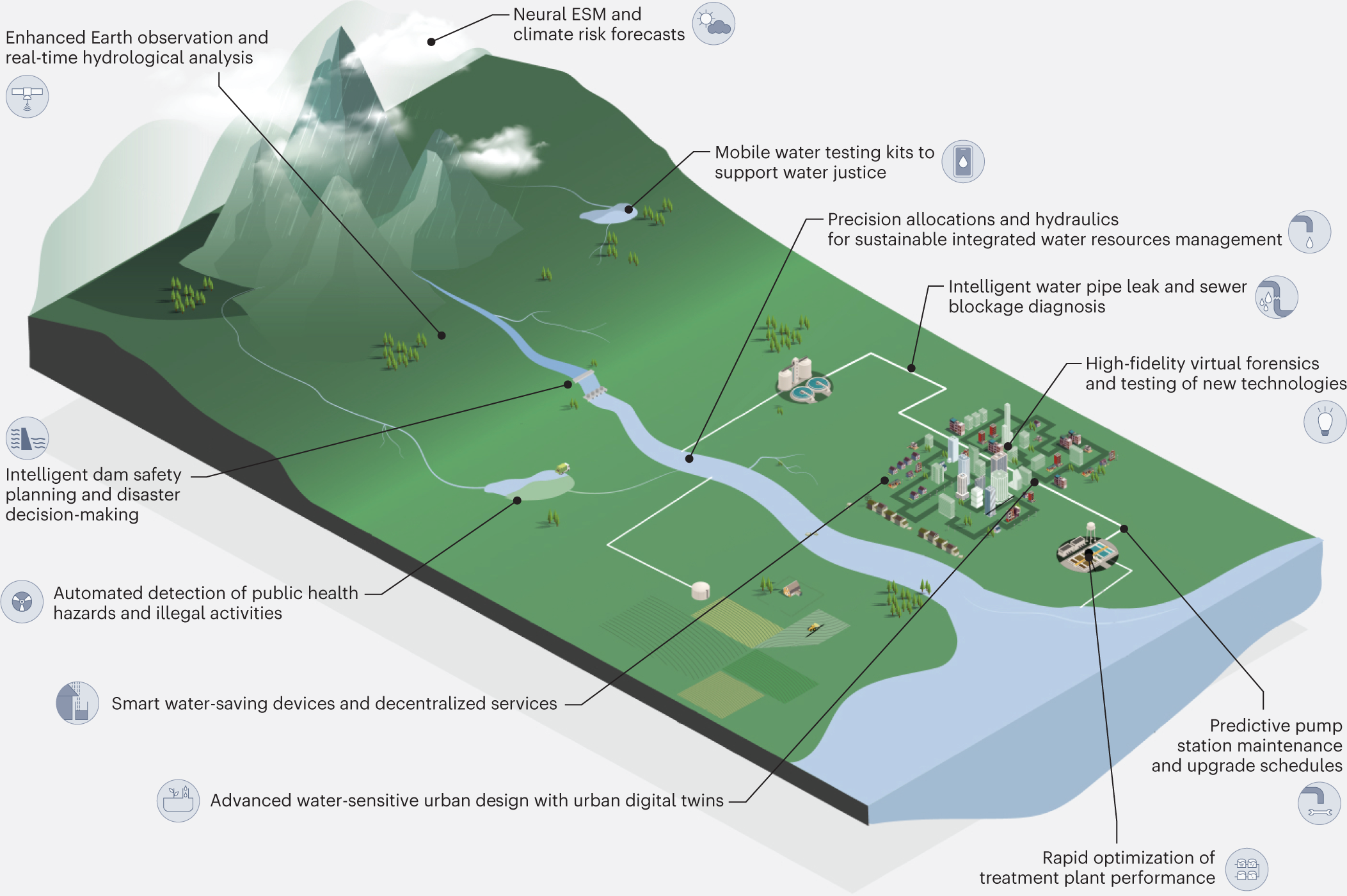The image is a detailed 3D illustrative diagram depicting a landscape model that integrates various aspects of environmental and resource management technology. Positioned diagonally from the top left corner to the bottom right corner, a green patch of land dominates the scene, surrounded by pertinent labels and annotations. Mountaintops adorned with white clouds—signifying "Enhanced Earth Observation and Real-Time Hydrological Analysis, Neural ESM and Climate Risk Forecasts"—anchor the top of the diagram. Below, water elements marked "Mobile Water Testing Kits to Support Water Justice," "Precision Allocations and Hydraulics for Sustainable Integrated Water Resource Management," and "Intelligent Water Pipe Leak and Sewer Blockage Diagnosis" occupy strategic points on the landscape, connecting to the blue-toned rivers and lakes. 

A large industrial building represents "High-Fidelity Virtual Forensics and Testing of New Technologies," while a cityscape icon highlights areas like "Predictive Pump Station Maintenance and Upgrades Schedules" and "Rapid Optimization of Treatment Plant Performance." The illustration, set against a pale gray background, also refers to urban development themes with labels such as "Advanced Water Sensitive with Urban Design and Urban Digital Twins" and "Smart Water Saving Devices and Decentralized Services." Additional features include "Automated Detection of Public Health Hazards and Illegal Activities" and "Intelligent Dam Safety Planning and Disaster Decision Making," emphasizing both technological innovation and environmental stewardship in a visually cohesive and informative manner.